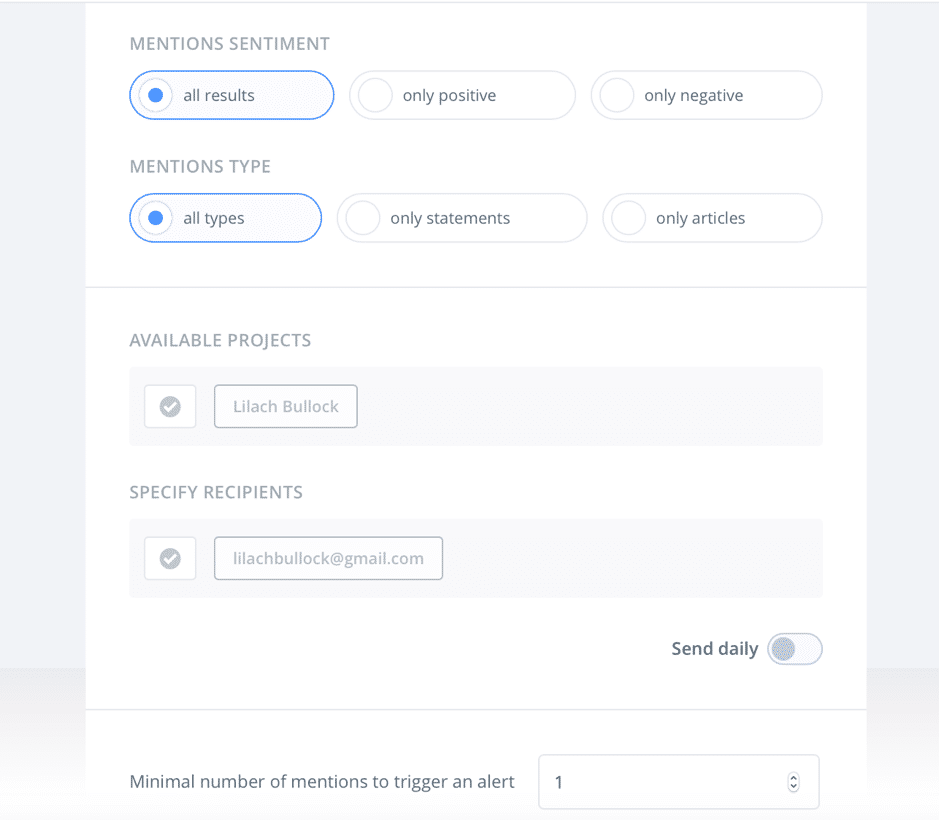This screen captures the search feature of a social media application, which is designed for tracking mentions across various platforms. The interface is framed by light blue vertical rectangles and features several options to customize the search parameters.

At the top, in a light blue font, is the section titled "Mentions Sentiment." Here, users can filter the results to display all mentions, only positive mentions, or only negative mentions.

Below this, the "Mentions Type" section allows users to narrow the search to show all types of mentions, only statements, or specifically articles.

In this scenario, the search is focused on mentions related to a person named Lilac Bullock. This is specified under the "Available Products" list. Users can further refine the search by targeting specific recipients; in this case, mentions are to be sent to the email address lilacbullock@gmail.com.

Additionally, there is a "Frequency" button, allowing users to set how often they want to receive updates. There's also an option to set a minimum number of mentions required to trigger an alert, ensuring that users are notified only when there is significant activity.